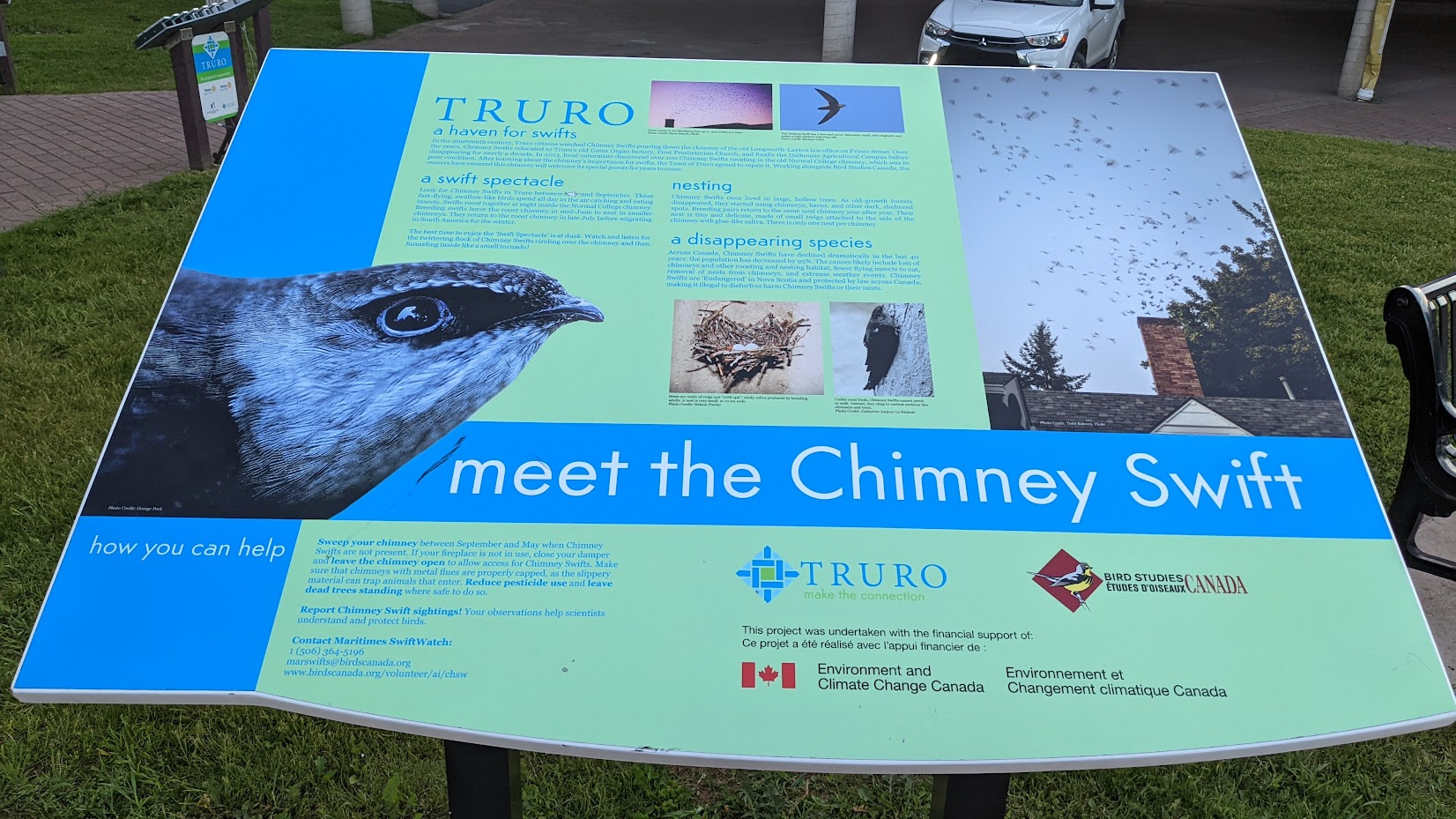This outdoor photograph, taken during the daytime, captures a well-detailed sign designed for a tourist area. The sign itself, approximately six inches wide and three inches tall, is mostly rectangular with a slight outward bowing at the bottom. The sign's left edge is adorned with a vertical blue banner where the head of a chimney swift bird is prominently featured in black and white. Adjacent to the bird's head, the text invites viewers to "meet the chimney swift" and informs "how you can help."

To the right of the bird's head, the blue banner extends horizontally, displaying the title "Meet the Chimney Swift" in white print. The right corner of the sign features an outdoor photograph of several chimney swifts flying either over or out of a chimney, adding a dynamic visual element. The background to the left and below the photograph is green, with blue text elaborating on topics such as "Truro, T-R-U-R-O," "A Haven for Swifts," "A Swift Spectacle," "Nesting," and "A Disappearing Species."

At the very bottom, the sign acknowledges its sponsors, including Truro, Bird Studies Canada, and Environment and Climate Change Canada, with the slogan "Make the Connection." The background setting includes a grassy park area, a parking spot at the top, a bench to the right, and a walkway with brick-like paving on the left, providing a serene and inviting atmosphere for park visitors.